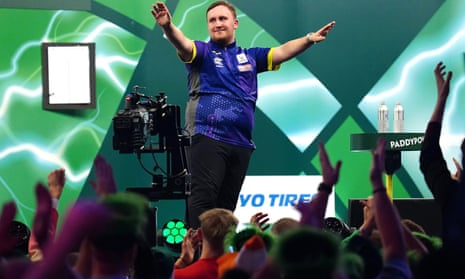The photograph captures a dynamic scene of a man standing on a stage with his arms outstretched, looking slightly towards his right. The man, who has short brown hair and appears to be a bit overweight, is wearing a blue t-shirt with yellow borders on the short sleeves and gray stripes down the sides, paired with black pants. He has a subtle smile on his face, indicating a celebratory or acknowledging gesture towards the audience. The background features a striking electronic pattern with various shades of green, blue, and white, resembling electricity or lightning stripes.

Below him, a diverse crowd is visible, with many individuals mid-clap and their hands raised, conveying enthusiasm and admiration. The crowd's energy is palpable, with the backs of their heads and expressive gestures prominently featured. To the man's left, a large black camera on a metal stand is positioned, likely capturing the event. On stage, a small table holds two large water bottles and a partially obscured sign that appears to read "Paddy Pop" or "Paddy Poe." Another sign below the stage, seemingly cut off, shows the text "VO tire" with blue font on a white background. The overall scene is vibrant, filled with colors like blue, green, black, yellow, gray, and white, and captures a moment of engagement and interaction between the performer and his audience.